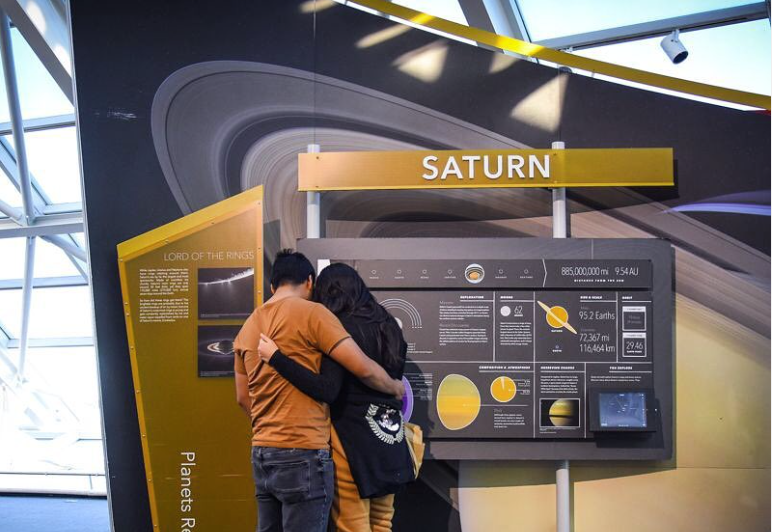In the image, a couple stands at the center of a science and technology museum, closely examining an exhibit about Saturn. They are positioned in front of a detailed astronomical chart displaying a dramatic photograph of Saturn, highlighted by its prominent yellow sphere and encircling rings set against a dark background. Above the chart, a vertical green bar with white text reads "Saturn," and beneath it, a larger board features illustrations and paragraphs of information about the planet. The man on the left, with black hair, wears an orange t-shirt and dark jeans, while the woman on the right, with long black hair, is dressed in a black sweater and orange pants. They stand with their arms around each other, heads closely tilted together. Natural light floods the museum through large windows in the background, casting a pleasant brightness over the scene. The colors in the image include various shades of orange, blue, black, beige, and tan.